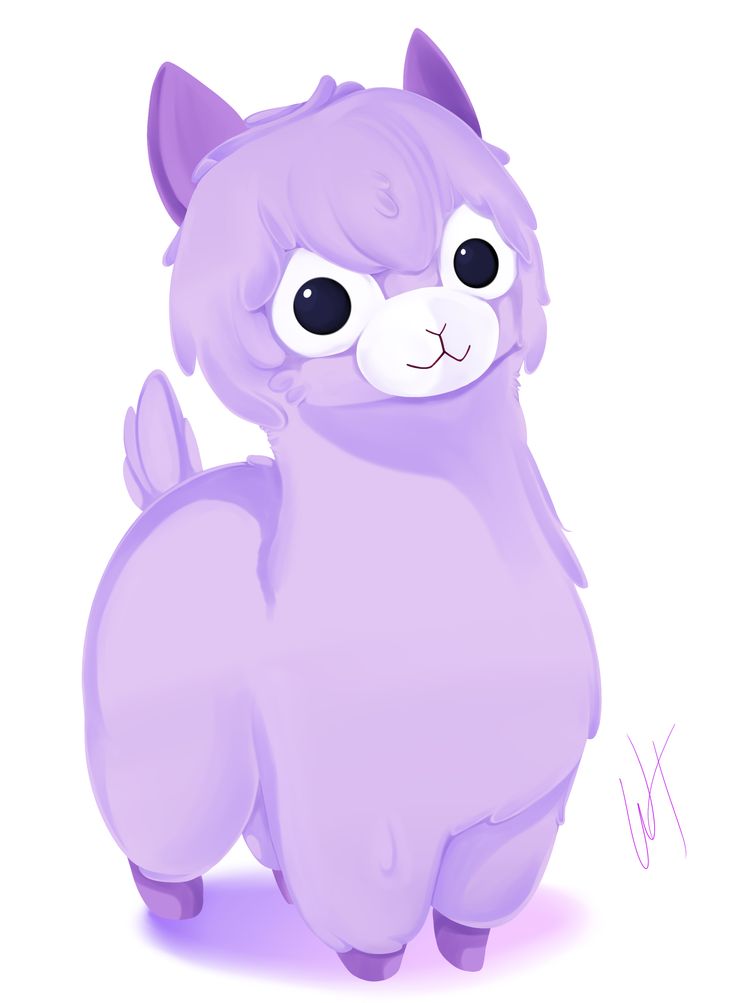This image features a cartoon-style depiction of a baby llama with detailed characteristics. The llama, standing in the center of the image, has light purple fur on its body and dark purple hooves. Its tail is elevated, and it has two dark purple ears standing upright on its head. The face is adorned with long hair, and it has two large, somewhat eerie white eyes with black centers. The nose is white with a dark purple outline, and the mouth is shaded purple. A signature with the letters "W" and "T" appears on the right side of the image. The overall appearance and color scheme suggest it might be a figure from a children's book or a toy, though there is no specific background to confirm the setting.